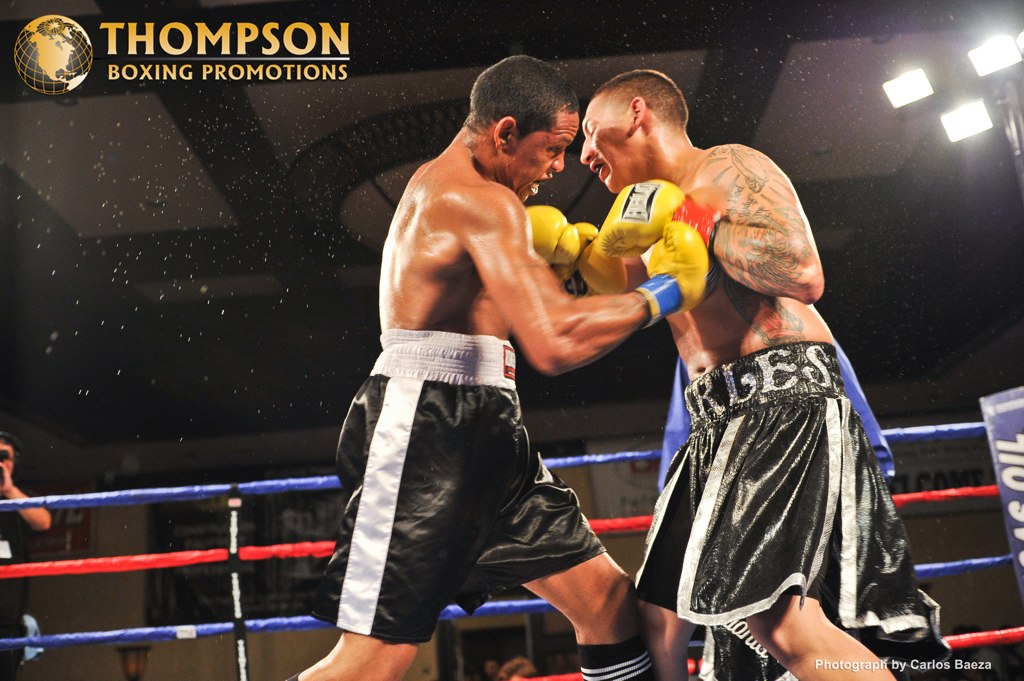The full-color promotional photograph captures an intense moment inside a boxing ring, where two fighters are engaged in heated combat at the center. Both boxers, one Caucasian and the other of potentially Hispanic or Black descent, sport very short cropped hair. They are outfitted in black trunks adorned with white stripes, though the designs differ subtly, and both wear striking yellow boxing gloves, a distinctive choice. The ring ropes are layered in a sequence of blue, red, and blue. Notably, a spray of sweat can be seen near the left of the left-side boxer, highlighting the intensity of the match. The dark ceiling contrasts with the bright lights illuminating the scene, specifically a yellow light in the upper right. In the left-hand corner, a logo of the world is visible, accompanied by the text "Thompson Boxing Promotions" in orange or yellowish color. The photograph, shot by Carlos Beza, functions as an advertisement for the boxing promotion, capturing the raw energy and physicality of the sport.